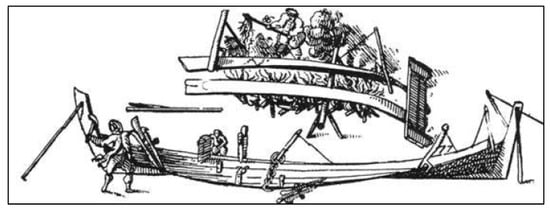This black-and-white illustration depicts a long rectangular scene of a wooden ship, approximately three times as wide as it is tall. The simplistic, hand-drawn image is divided into two main portions. The bottom section features a long boat driven by oars, notable for its lack of sails. Surrounding the boat, there appear to be several figures: on the far left stands a person who might be wielding a tool, weapon, or shield, possibly involved in the construction or defense of the vessel. Another figure seems to be kneeling on the boat, while other indistinct parts and pieces of the ship are scattered around. 

The top portion of the illustration portrays a chaotic bridge-like structure where people stand, some seemingly shooting down towards the boat below. This upper scene is characterized by a jumbled array of lines creating a sense of disorder. Both the top and bottom parts of the image are interconnected by these activities, as if depicting an ongoing interaction or event. The overall image is framed by a clean black border, highlighting its stark, monochromatic aesthetic.